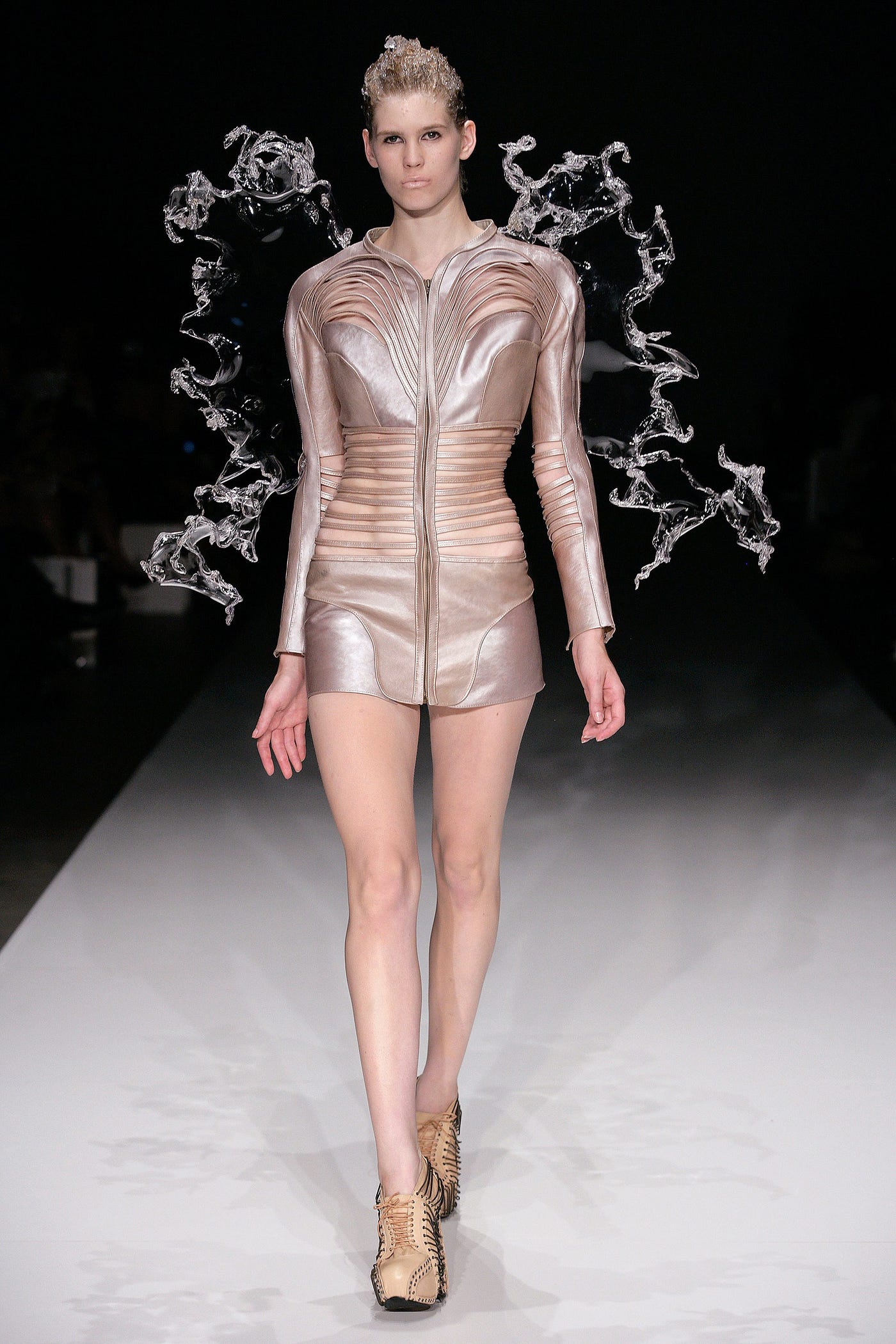A striking fashion model stands on a sleek gray runway, enveloped in an aura that blends realism with the uncanny. The male model’s short hair is meticulously styled into an upward updo, giving an edgy complement to his bold look. He wears an unconventional, futuristic long-sleeved mini dress that tapers to the upper thigh. This dress appears to be made from a leather-like material with a silvery-gray satin sheen, and features intricate cutout designs—striped around the midriff and forming rounded arches over the décolleté and shoulders, providing glimpses of bare skin.

The model's legs are visibly bare, accentuating his tall, statuesque frame. His tan shoes, designed with a striped motif and darker brown accents, anchor his outfit whilst adding subtle contrast. A mesmerizing, almost ethereal element is present: what appears to be flowing water caught in mid-motion emanates from his back, resembling either clear plastic wings shaped to mimic water or an actual splash of water frozen in time by a camera flash, enhancing the snapshot with a sense of dynamic fluidity. This accessory, possibly mimicking wings, reinforces the futuristic and avant-garde theme of the ensemble.